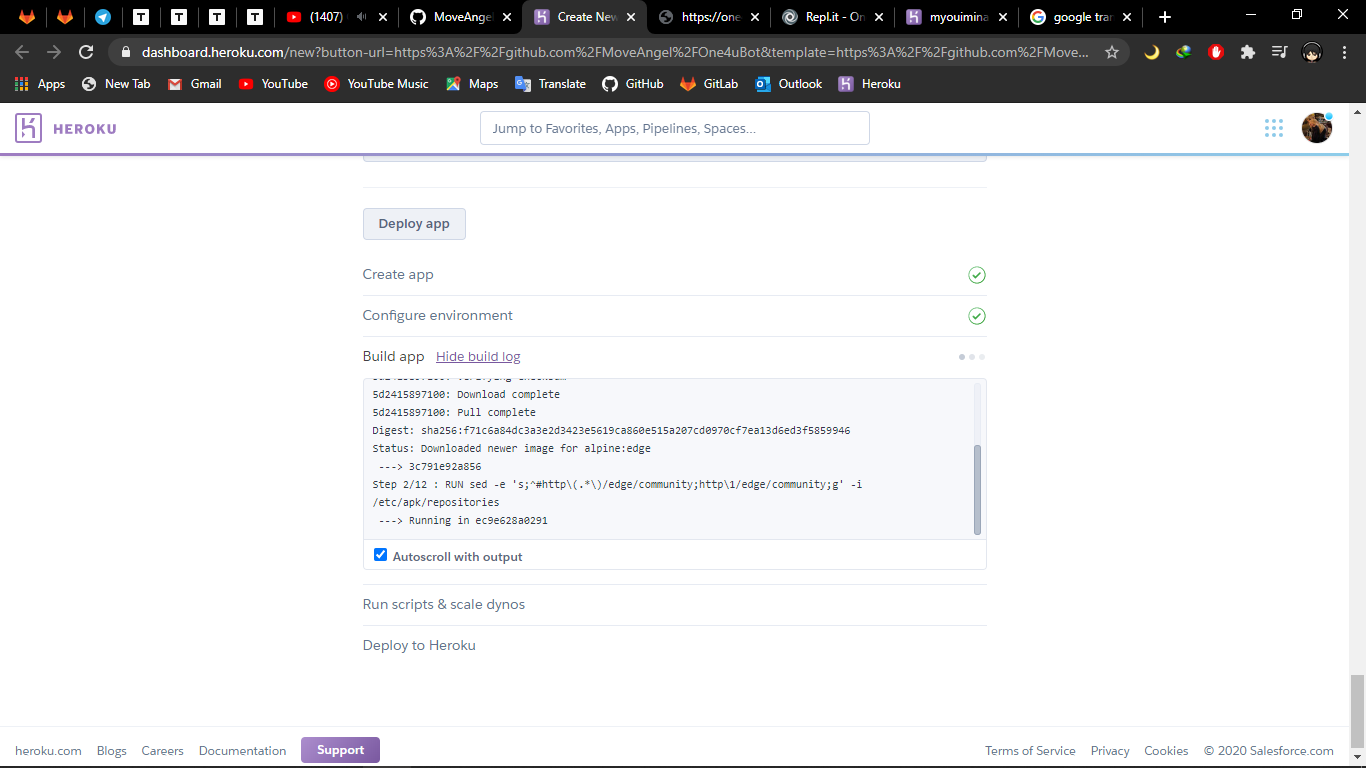The image is a screenshot from a computer screen, potentially from either a desktop or a laptop. The screenshot captures a web browser in dark mode, with the tab bar at the top in black and the address bar and bookmarks bar in dark gray. The user is viewing the website dashboard.heroku.com. The page features a white background. In the upper left-hand corner, there is a purple logo consisting of a lowercase "h" inside a square. Beside the logo, the text "HEROKU" is written in uppercase letters. Below the logo, there is a search box with the placeholder text "Jump to favorites, apps, pipelines, or spaces," indicating that the user can type in it to navigate to different sections. Further down the page, there is a box displaying black text in a monospaced font, resembling code typically seen in a command line interface.